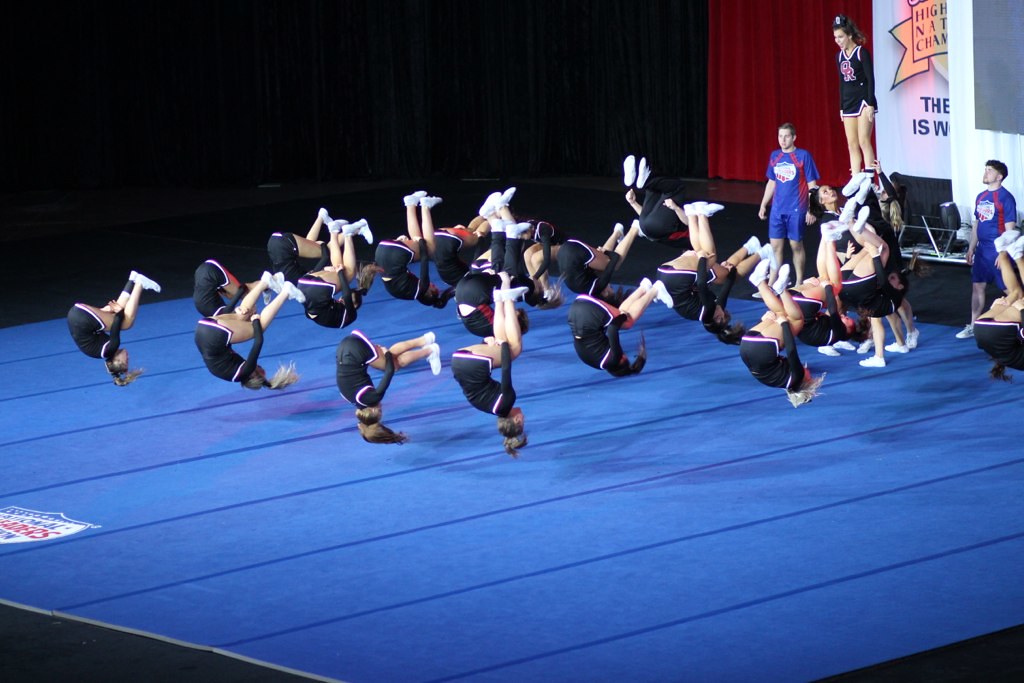The image captures a vibrant scene inside a large auditorium, possibly a theater or stadium, during a high school national championship cheerleading competition. Against a mostly black background, the stage is a striking blue floor adorned with darker blue lines and a logo on the left-hand side. Dominating the center, a group of cheerleaders, dressed in dark blue uniforms with red and white stripes, is captured mid-backflip, each frozen in an upside-down moment. To the right, a red curtain partially frames the scene, where a woman stands observing the performance. At the front of the stage are two men in blue and red jerseys, sporting an American-like shield emblem. A sign in the background, slightly obscured, reads 'Hi Nat Cham,' hinting at the High School National Championship event. Additionally, a blue rectangle is visible on the far right-hand side, completing the lively and dynamic composition.